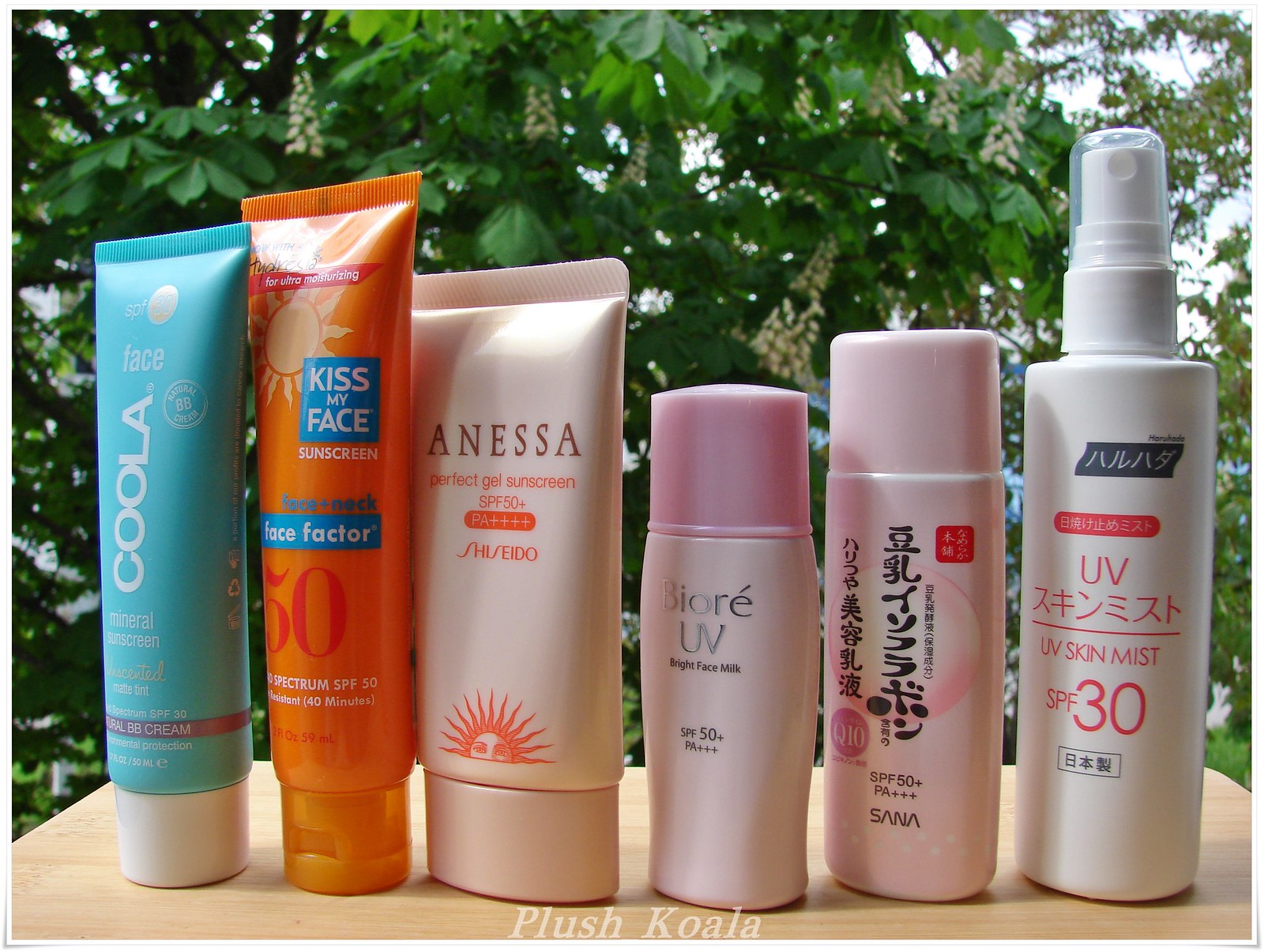The image features a row of seven beauty products neatly lined up on a table set against a verdant background of lush, broad-leaved trees. Clearly taken outdoors, the photograph captures each item in detail. Starting from the left, the first product is a blue face care item named "Kula." Next to it is an orange tube labeled "Kiss My Face."

The third item, from "Vanessa Shiseido," is followed by the fourth, which is from "Biore UV." This Biore UV product stands out as the smallest and shortest in the lineup, characterized by its unique shape resembling a deodorant. It features a pastel pink body, a pink cap, and is clearly labeled as SPF 50, indicating it's a facial lotion.

The fifth product is pink and bears Chinese characters, with additional markings indicating SPF 50+ and "SA, NA" at the bottom. Completing the row on the right is a spray bottle with a clear cap and a white body, adorned with Chinese characters. The only English found on this item is "UV Skid Mist SPF 30," suggesting it provides sun protection. 

This well-curated selection of beauty products is captured in a serene natural setting, emphasizing both diversity and attention to detail.